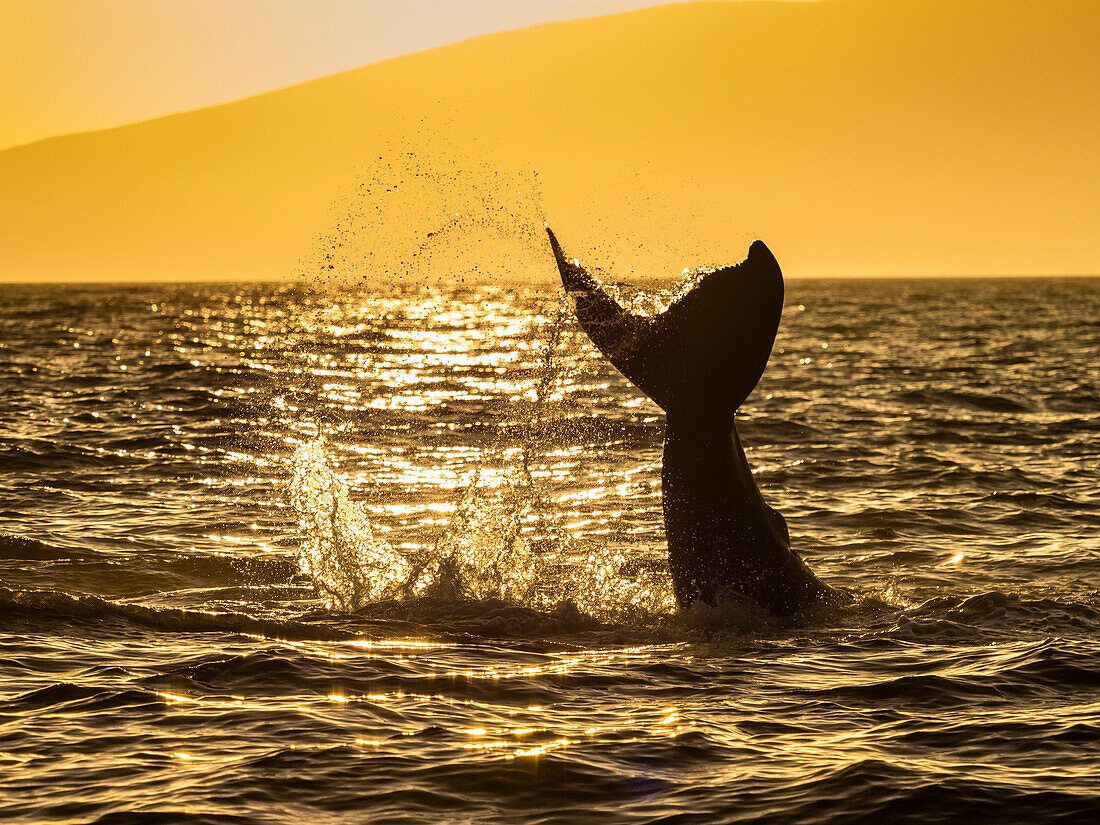The image depicts a majestic scene of a large whale gracefully flipping its massive tail up in the air. As the sun sets, the sky takes on a brilliant yellow hue, transitioning to a lighter, almost pinky-beige shade in the top left corner. The softly shimmering sunlight creates a sparkling effect on the surface of the water, making subtle waves and turning the water a strange shade of gray. The silhouette of the whale's tail, striking in its heart-like shape, stands out in sharp contrast as a dark, black form against the colorful sky. Water splashes around the tail, adding dynamic motion to the serene environment, while the shimmering reflections of the sun dance on the water's surface. The overall composition highlights both the immense size of the whale and the tranquil beauty of its natural habitat.